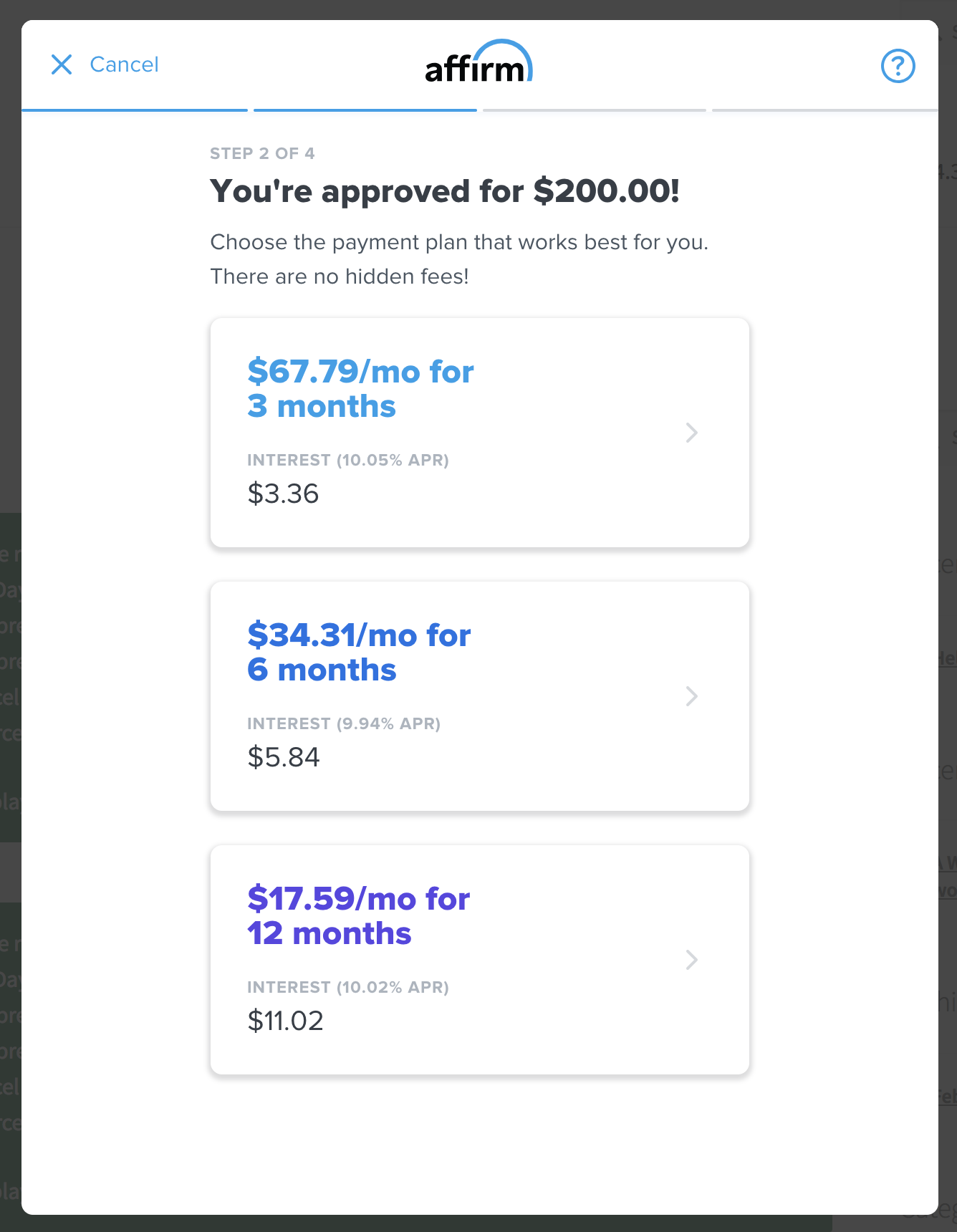This image is a screenshot from the website Affirm, showcasing the progress a user is making through a multi-step process. The user is currently on step two out of four. In the upper left-hand corner, there's a blue "X" followed by the word "Cancel." At the top center, the Affirm logo is prominently displayed. On the upper right-hand corner of the screen, there's a question mark icon.

The screen reads "Step 2 of 4: You are approved for $200. Choose the payment plan that works best for you. There are no hidden fees." Below this message, three different payment plan options are detailed:

1. The first plan is $67.79 per month for 3 months with an interest rate of 10.05% APR, resulting in $3.36 of interest.
2. The second plan, positioned in the middle, is $34.31 per month for 6 months with an interest rate of 9.94% APR, resulting in $5.84 of interest.
3. The third plan is $17.59 per month for 12 months with an interest rate of 10.02% APR, resulting in $11.02 of interest.

Each payment plan is clearly outlined, providing the monthly payment amount, the interest rate, and the total interest. The screen is outlined with a thin black border, and it appears to overlay another webpage, suggesting this is a pop-up window. 

Above the payment plans and below the "Cancel" button and Affirm logo, there are progress banners. The first and second steps are highlighted in blue, indicating completion, while the third and fourth steps remain gray, indicating they are still pending.

The overall layout is designed to guide the user through the selection of a payment plan with clear, essential information prominently displayed.